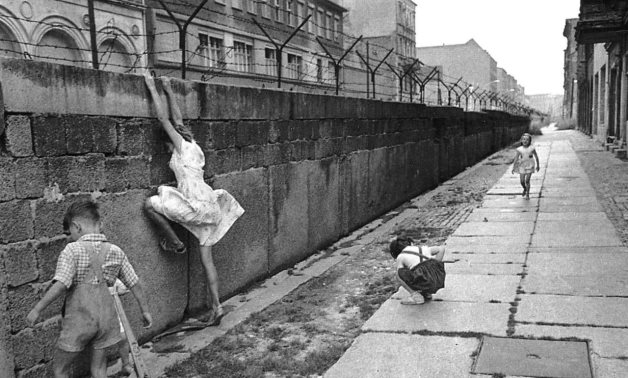The black-and-white photograph depicts a drab, concrete sidewalk adjacent to towering, old, and rundown buildings. A young girl in a dress attempts to scale a stone and concrete wall topped with Y-shaped barbed wire posts, indicative of a possible prison or historical landmark like the Berlin Wall. She reaches for the top of the wall, her foot precariously balanced on the rough surface. Surrounding her are three barefoot children wearing shorts – one boy and two girls – who stand close by, with their backs turned to the viewer. Farther down the narrow walkway, another girl faces the camera from a distance. The sky appears overcast, casting a somber tone across the scene, which is accentuated by the weeds sprouting through the cracks in the sidewalk.